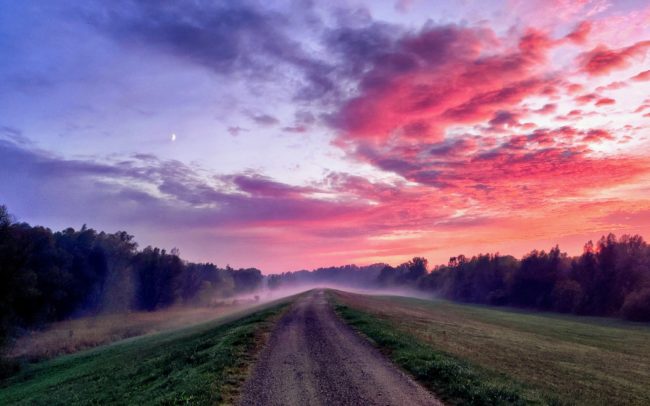This evocative image captures a single-lane country road stretching into the distance, perched atop a gentle hill. Flanking the road are well-maintained grassy fields that seamlessly transition into dense forests on either side, creating a natural corridor. The scene is bathed in the soft, twilight glow of the setting sun, casting the sky in a mesmerizing tapestry of pink, red, purple, orange, and blue hues. Enhancing the dreamy quality of the photograph, a thin film of mist and fog rises from the ground, giving it a hazy, ghostly ambiance. Amidst the colorful sky, a glimpse of the moon can be seen, adding to the surreal beauty of the moment. The unique combination of elements – the serene landscape, the vibrant sunset, and the ethereal mist – makes this visually striking and memorable.